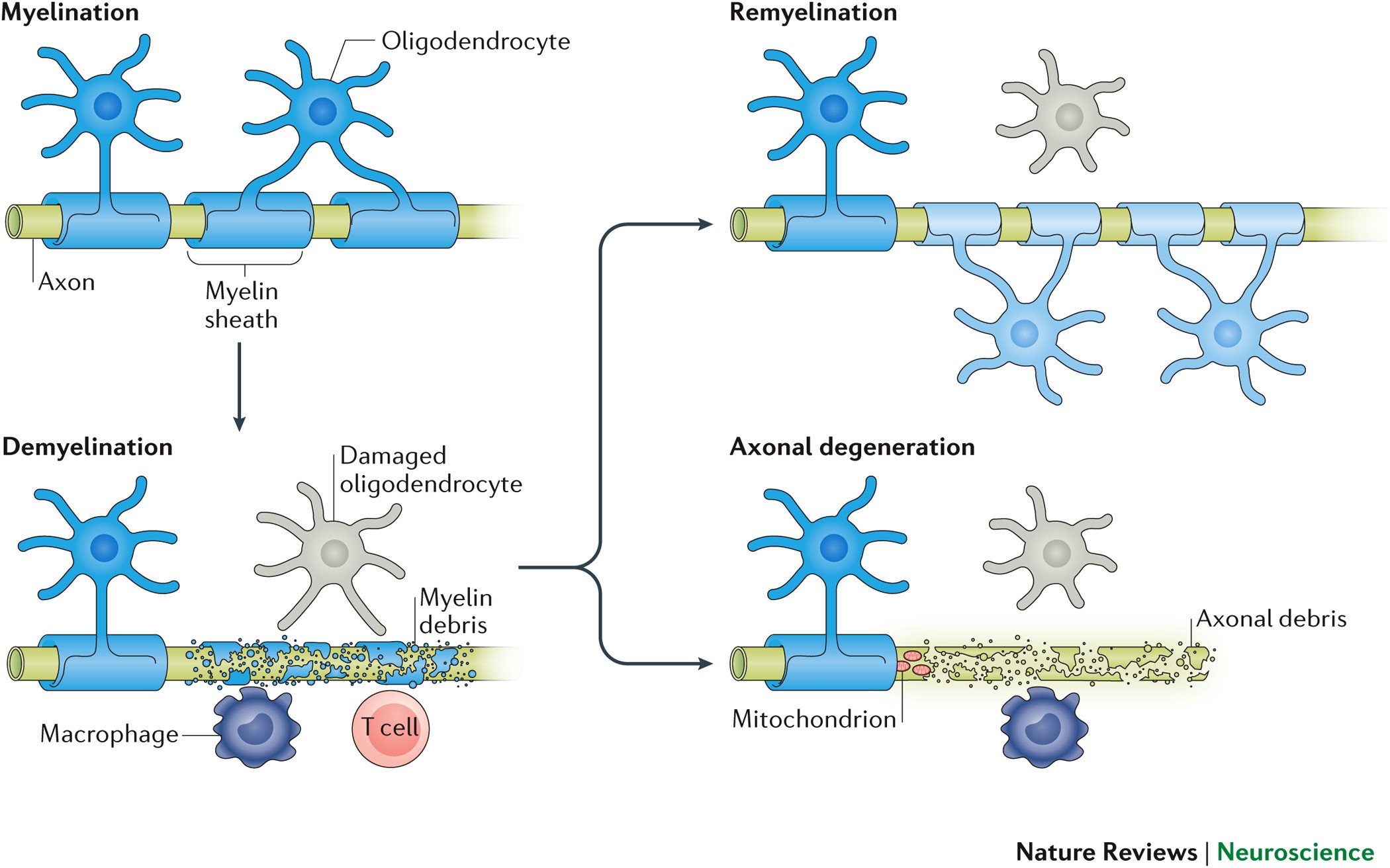The image is a detailed scientific diagram featured in *Nature Reviews Neuroscience,* depicting the process of myelination, demyelination, and the subsequent effects on axons. At the top left, the diagram starts with the myelination process, showing a green axon encased in three blue myelin sheaths formed by oligodendrocytes. The myelin sheaths appear segmented by blue tentacled balls labeled as oligodendrocytes. Moving down, the diagram illustrates demyelination, where the same green axon now shows damage with broken myelin debris along its length. Here, a purple circle labeled macrophage and a red circle labeled T-cell indicate the immune response, while a damaged oligodendrocyte is depicted nearby. Arrows lead from this stage to two possible outcomes: remyelination and axonal degeneration. In remyelination, the green axon begins to show partial regrowth of the myelin sheaths. In contrast, axonal degeneration is depicted with the disintegrating axon and resultant axonal debris. This comprehensive diagram helps visually summarize the cellular and molecular changes involved in nerve damage and repair processes relevant to neuroscience.